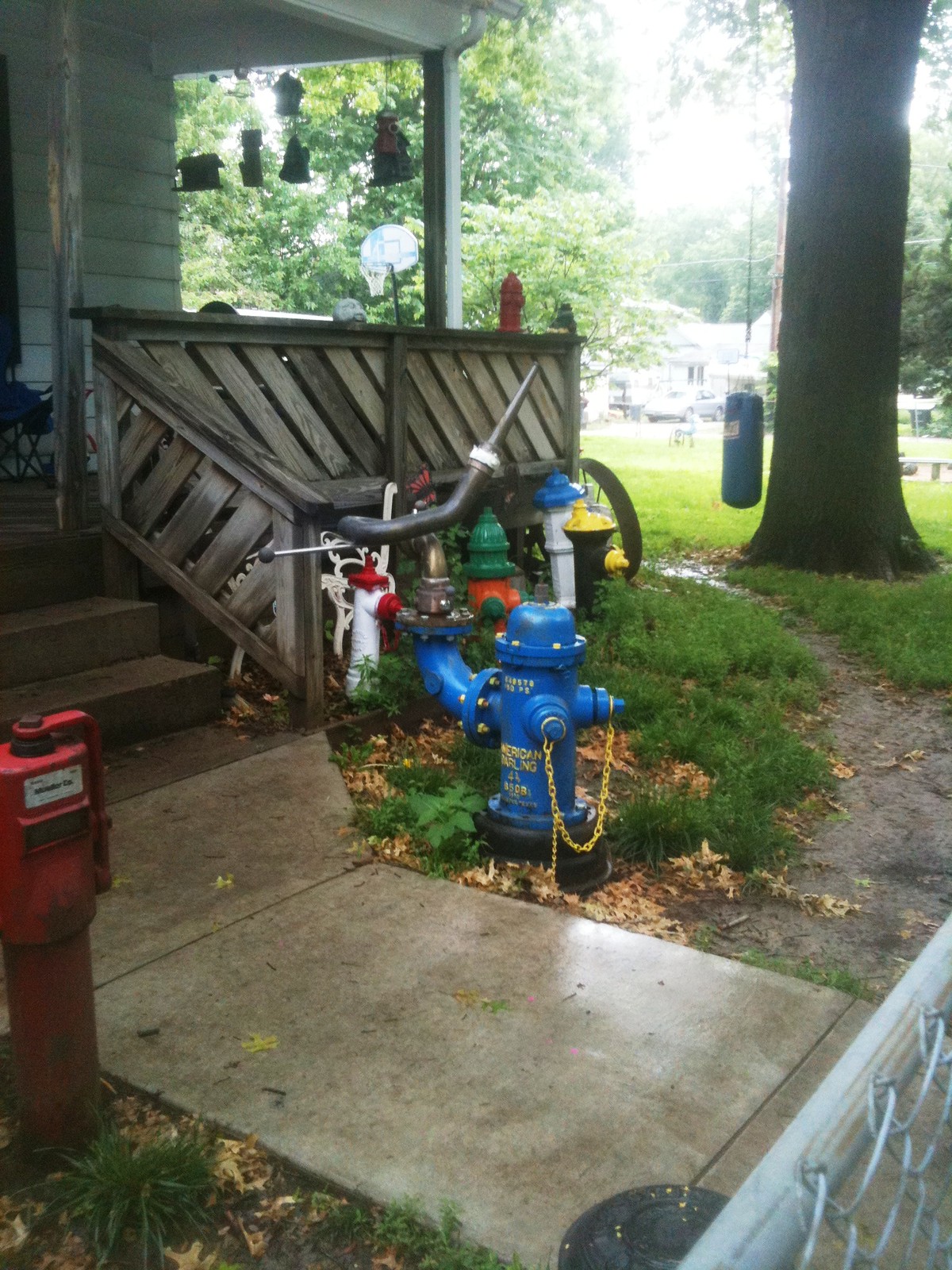This is a detailed portrait-style photo of a suburban home's front yard, showcasing an array of colorful fire hydrants. Prominently featured in the foreground is a blue hydrant with a complicated pump apparatus attached to it, accompanied by several other hydrants in various colors including red, white, orange, green, and black. They are arranged on a worn grassy patch next to a concrete sidewalk that leads up to a few concrete steps and a wooden porch with plain wooden railings reminiscent of a beach pier. Hanging from the porch are several bird feeders. Off to the right, a large tree with a wide trunk hosts a blue punching bag suspended from one of its sturdy branches. Scattered leaves on the ground suggest it might be fall. In the background, additional suburban houses are visible, completing the serene, tree-lined neighborhood scene.